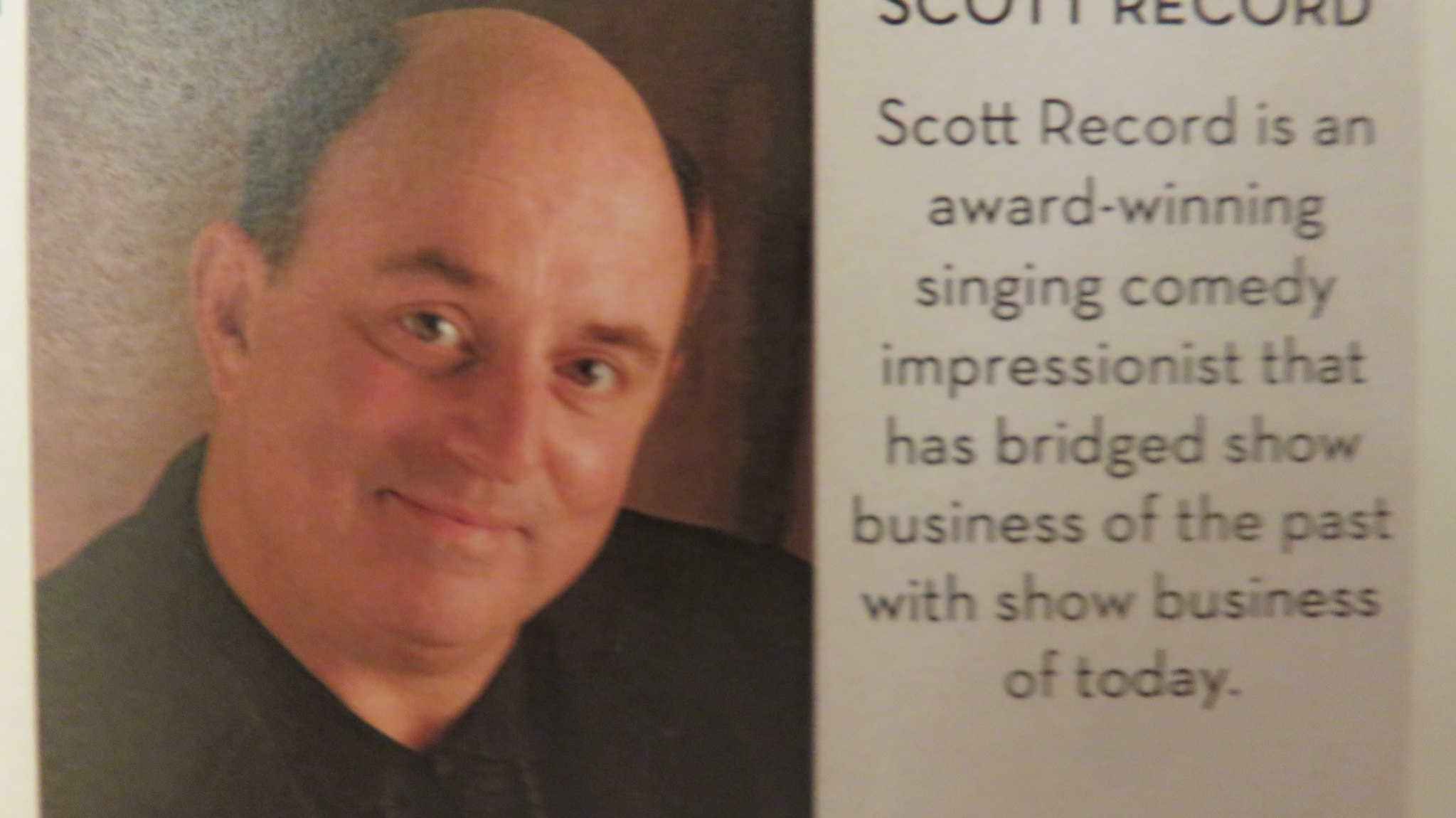The image features a horizontal rectangular photo business card. The left side of the card contains a headshot of a middle-aged Caucasian man named Scott Record. He has a balding head with brownish-gray hair on the sides and sand-colored eyebrows. He is slightly smiling with his mouth closed, and his light brown or hazel eyes have a few lines under them. His head is slightly tilted to the right, and he has minimal facial hair, with just some light stubble around the mustache area. He is dressed in a black button-up shirt paired with a black jacket. The background behind him includes a stone wall on his left and a wooden or dark wall on his right. 

The right half of the card has a buff beige-colored background with black text. The top line, partially cut off, reads in capital letters, "Scott Record." Below, in center-justified upper and lowercase letters, the text describes Scott Record as "an award-winning singing comedy impressionist that has bridged show business of the past with show business of today." The description takes up the right half of the view.